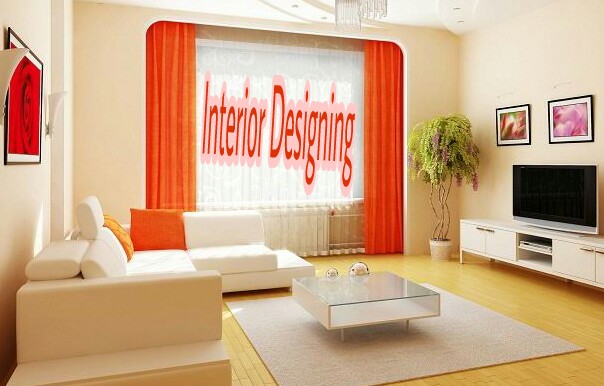This photo features a bright, predominantly white living room with a modern interior design. The room is centered around an L-shaped sectional couch, which is accessorized with bright orange throw pillows. The walls and cabinets are white, with the wall opposite the TV featuring a striking red painting. A large television sits on a sleek TV stand, beneath two vibrant pictures. The flooring is a light wood stain, mostly covered by a beige area rug that sits under a small glass coffee table. The window, dressed in bright orange curtains that match the pillows, bears the words "Interior Designing" in the same hue, suggesting it's an advertisement for an interior design company. A plant in a white pot adds a touch of greenery in the corner, complementing the overall bright and airy ambiance of the room.